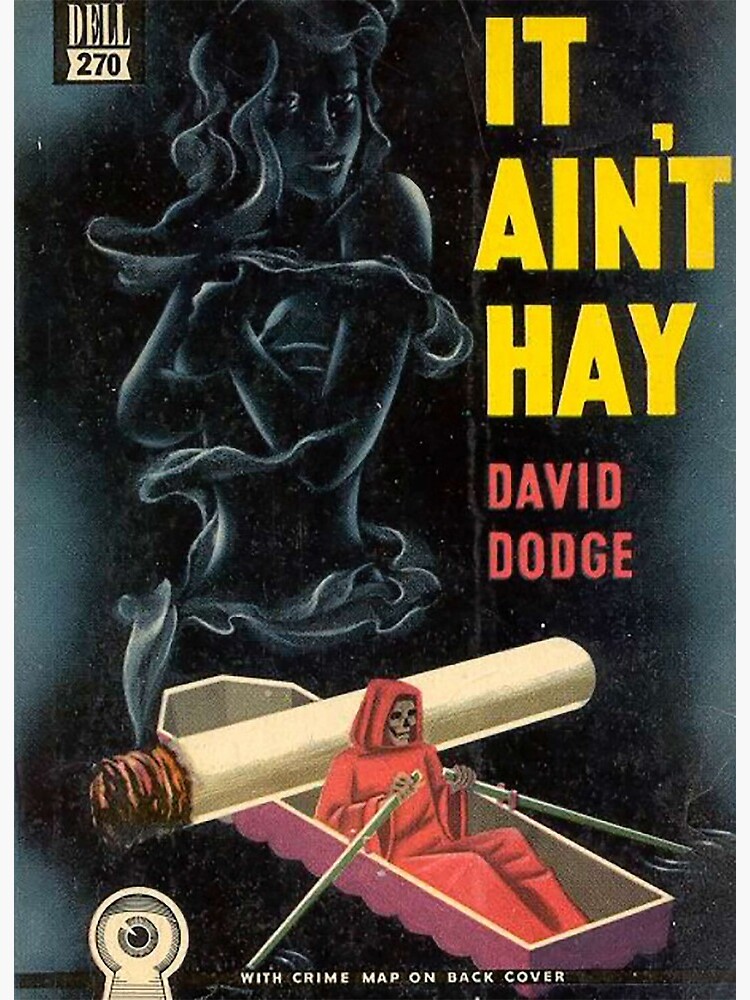This illustration, likely a book cover, features a striking graphic set against a dark black background. In the top left corner, a small box displays the text "Dell 270." Dominating the scene is a wispy, ethereal figure of a woman, seemingly made of smoke, which twirls around her body and forms her hair, with a serene smile on her face and her arms covering her breasts. Adjacent to this smoke figure, bold yellow letters declare the title "It Ain’t Hay," and below that, the author's name "David Dodge" appears in red.

Just beneath this central illustration is a grim yet intriguing scene: a coffin shaped like a boat, which is being rowed by the Grim Reaper dressed in a striking red robe. The Grim Reaper’s hands clutch two oars, steering the coffin-boat through an unseen body of water, while an oversized lit cigarette rests across the back of the coffin, its smoke seamlessly forming the image of the woman above. At the bottom of the cover, an eyeball within a keyhole suggests a hidden perspective, accompanied by the text "With crime map on back cover."